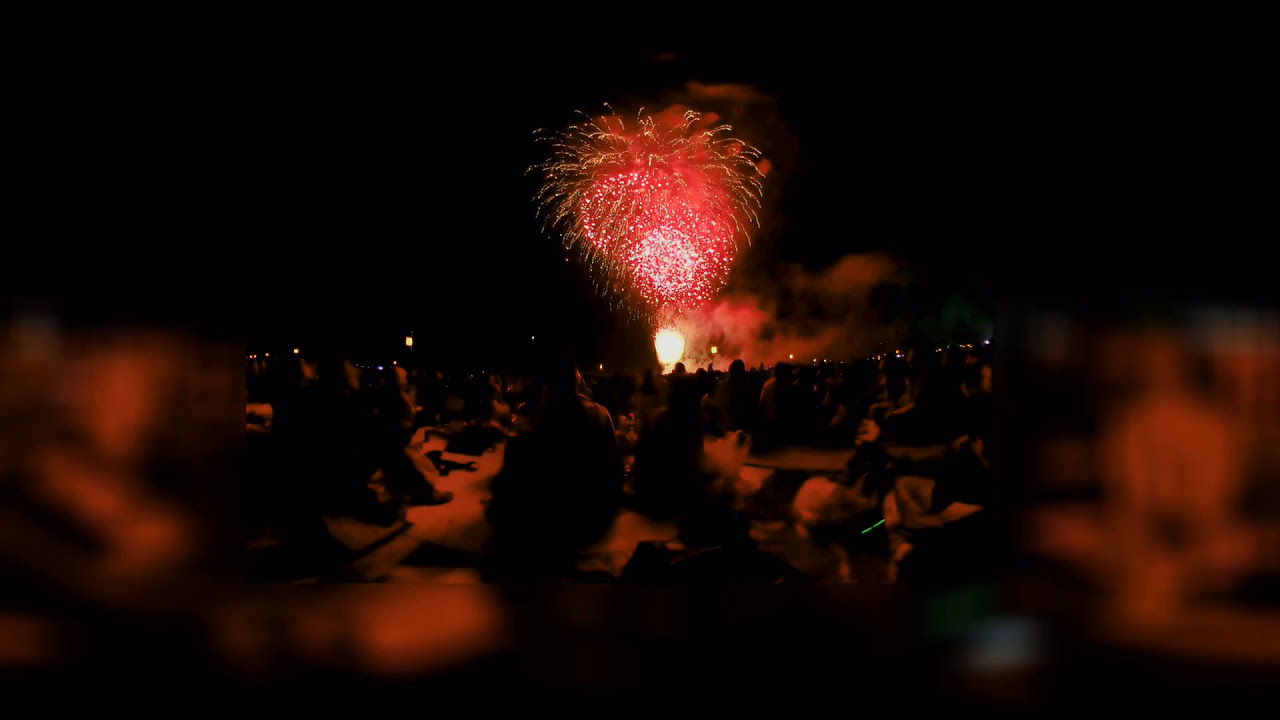In this nighttime photograph, a large crowd of people is sprawled on the ground, closely gathered and watching a firework display. The scene is dominated by darkness, with only the light from the fireworks breaking through the black sky. In the center of the frame, a single firework bursts, emitting glowing red tendrils, while faint smoke from previous fireworks lingers in the background. The display seems unusually low to the ground, accentuating the potential danger from the firework's proximity. To the right, a young person stands out, holding a glowing wand, possibly adding her own touch of light to the spectacle. The overall ambiance is muted and blurry, yet it crisply captures the essence of a communal firework celebration under a darkened sky.